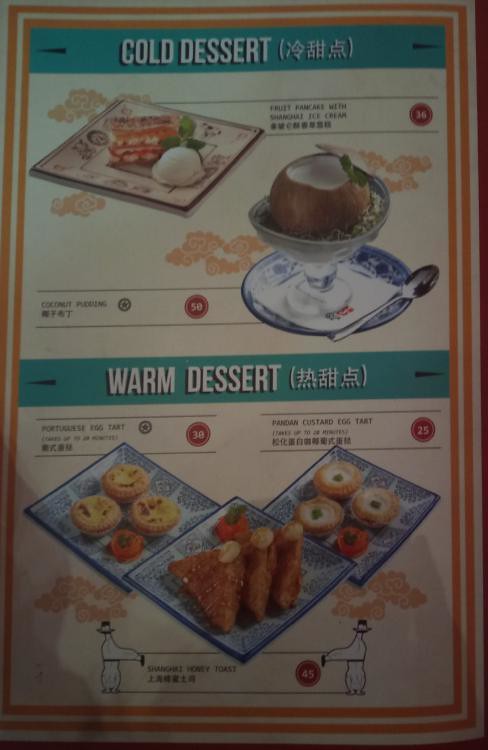The image is a photograph of a Chinese restaurant menu, featuring distinct sections for both "Cold Desserts" and "Warm Desserts," with descriptions in both English and Chinese. The menu is framed by a yellow and white border, with blue header borders for each section. The top section, labeled "Cold Desserts," includes visually appealing photographs of various desserts, such as an intricately plated dish with a scoop of white ice cream accompanied by a pinkish element and decorative leaves. Among the cold desserts, there's also a specific image of a coconut dessert served in a clear glass dish, with the number "50" marked beside it. The pricing and additional descriptive text are in Chinese.

The lower section, labeled "Warm Desserts," showcases items like egg tarts and custard egg tarts, each displayed on blue-rimmed plates. Notable mentions include "Portuguese Egg Tart" and "Shanghai Honey Toast," although the text is somewhat blurry. The layout is enhanced with flower designs on both sides, adding a decorative touch to the otherwise white menu. Some numbers, such as "36" circled in red, appear alongside certain desserts. Overall, the menu provides a blend of beautifully plated desserts along with partially legible pricing and descriptions, primarily in Chinese.